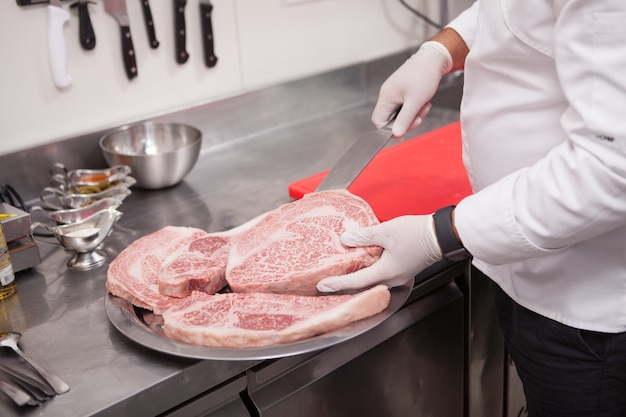The image depicts a professional kitchen where a chef, whose face is not visible, is the focal point. The chef stands at the right edge of the frame, wearing a white chef's jacket, black pants, white gloves, and a black wristwatch on the left wrist. He is holding a large knife in his right hand and is in the process of handling one of four large cuts of raw steak on a silver platter with his left hand. The work surface is a stainless steel countertop, accentuated by a red cutting board positioned nearby. Five small stainless steel gravy boats, each containing different sauces—white, red, and green among them—are aligned on the counter. To the left, a cluster of spoons and other silver utensils are partially visible. In the background, six knives with various handle colors, including one with a white handle, are mounted on the white wall, adding to the professional ambiance of the kitchen. The overall scene emphasizes the meticulous and organized environment where the chef is presenting the meat.